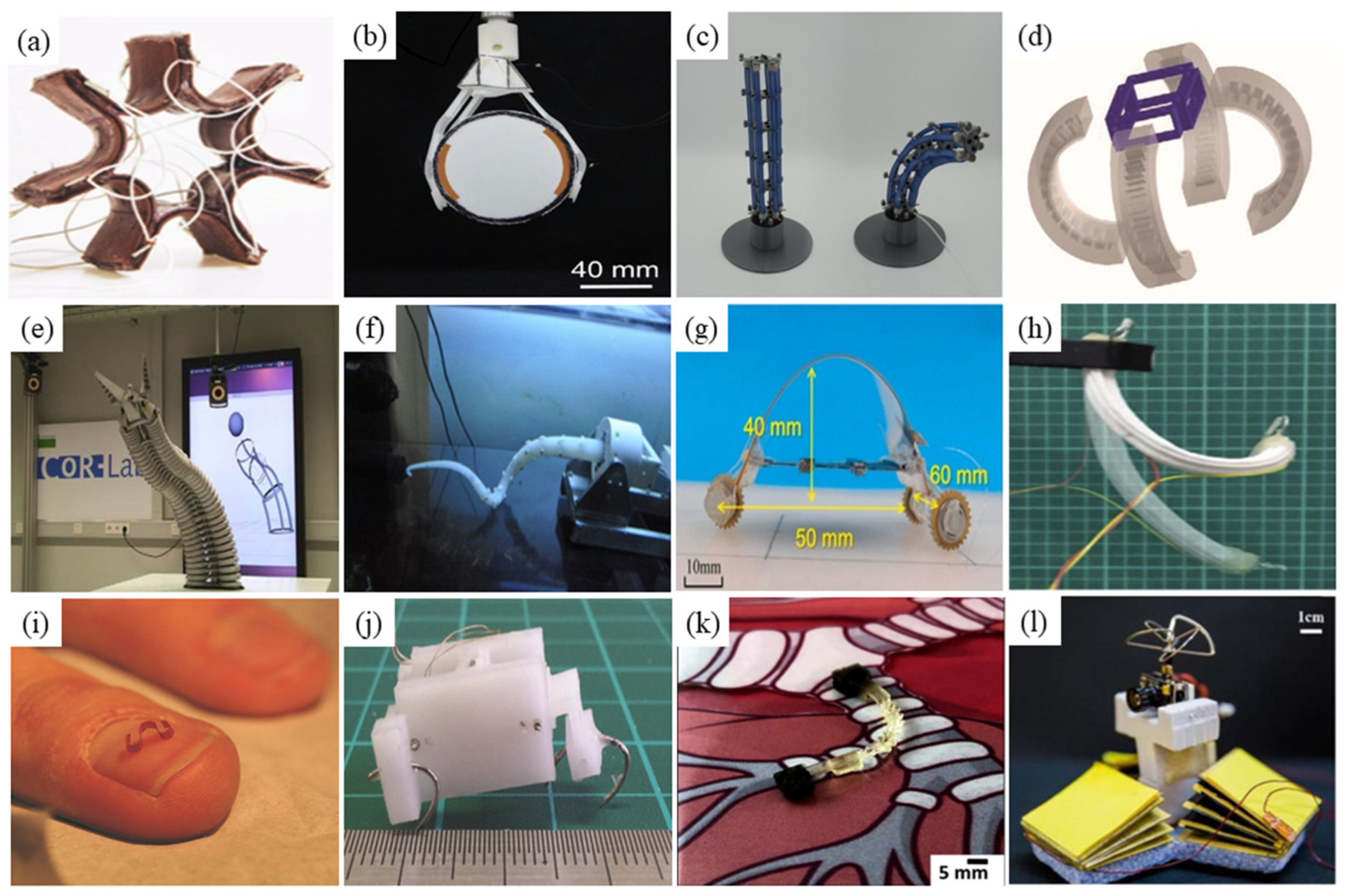The image is a detailed chart organized into a 4x3 grid, containing 12 labeled thumbnails from A to L. Each thumbnail showcases various technological and engineering devices, with a focus on miniature and complex machinery. Starting from the top left, Thumbnail A involves circuits, while Thumbnail B features a machine which is marked "40mm" at the bottom right. Thumbnails C and D are unclear. Thumbnail E shows a device in front of a screen, and Thumbnails F, G, and H depict more intricate machinery. Thumbnail I, located at the bottom left, displays a close-up of two fingers, with a tiny object placed on the middle fingernail. The last row contains electrical equipment in Thumbnails J, K, and L, aligning with the overall theme of advanced technology and miniaturization.